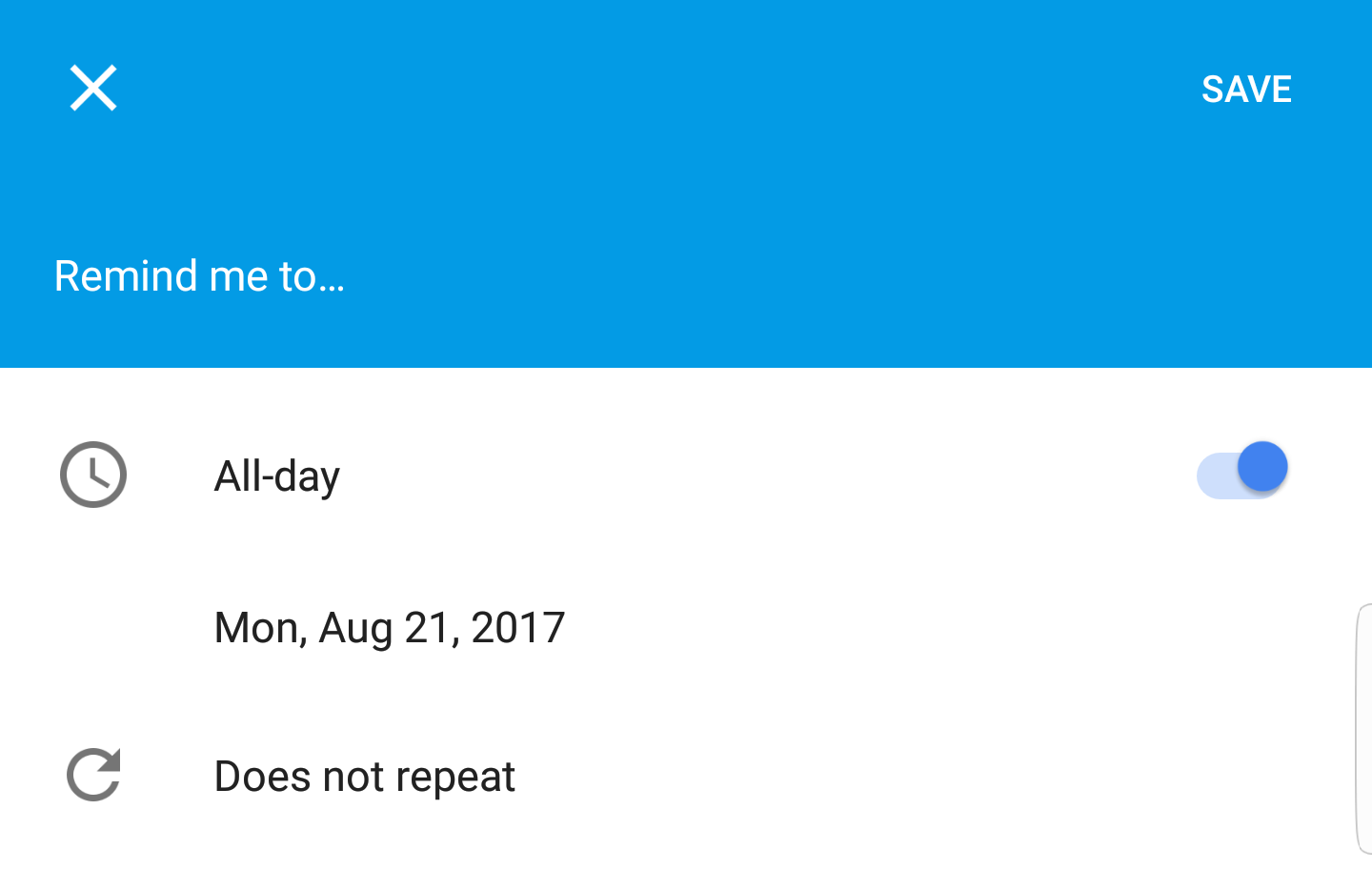This website features a minimalistic and straightforward design with a predominantly white background. At the top, there's a large blue box with a centrally located white X in the upper left-hand corner. The word "SAVE" is prominently displayed in capital letters in the upper right-hand corner of the blue box. Below this box, in the bottom left corner, the text "REMIND ME TOO..." is visible, while the lower right corner remains blank.

An image of a black clock is situated within the content area, indicating "ALL DAY," which is highlighted in blue, signifying that this setting is active. The date "MONDAY, AUGUST 21st, 2017" is prominently displayed, followed by a near-complete circular arrow symbol indicating "DOES NOT REPEAT."

On the right-hand side of the page, there is a light gray partial image with a vertically oriented line running through its center, and the top and bottom edges of this image are rounded. The page concludes with no additional elements, maintaining a clean, white background throughout.